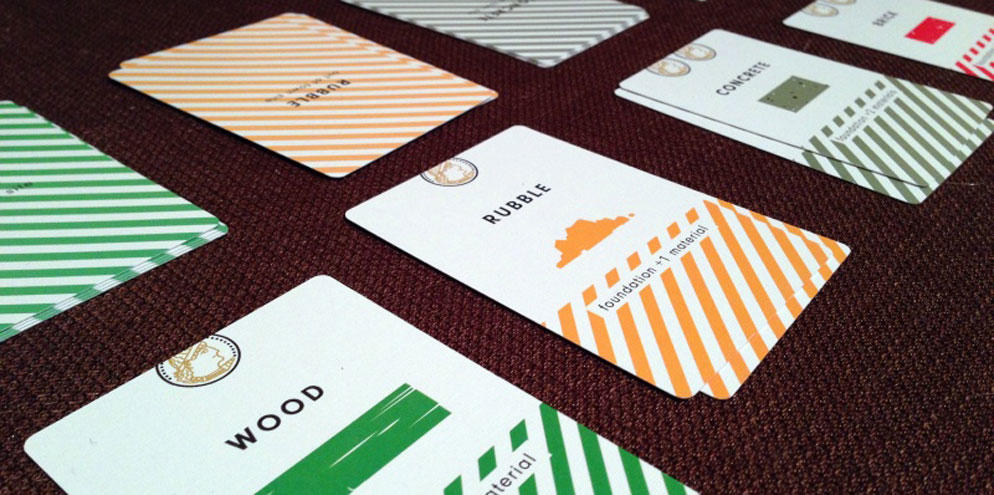The image depicts a card game in progress on a textured burgundy tablecloth. Four rows of cards are visible: face-down decks on the left and face-up cards on the right. Each face-up card displays a different material and corresponding colored stripes. The green-striped card says "wood," the orange-striped card says "rubble," the gray-striped card says "concrete," and the red-striped card says "brick." The cards are lined up neatly, with illustrations and text indicating "foundation +1 material." Some cards have an insignia resembling a person's face turned to the side. The composition shows a well-organized game setup, hinting at a unique and unfamiliar card game involving construction materials.